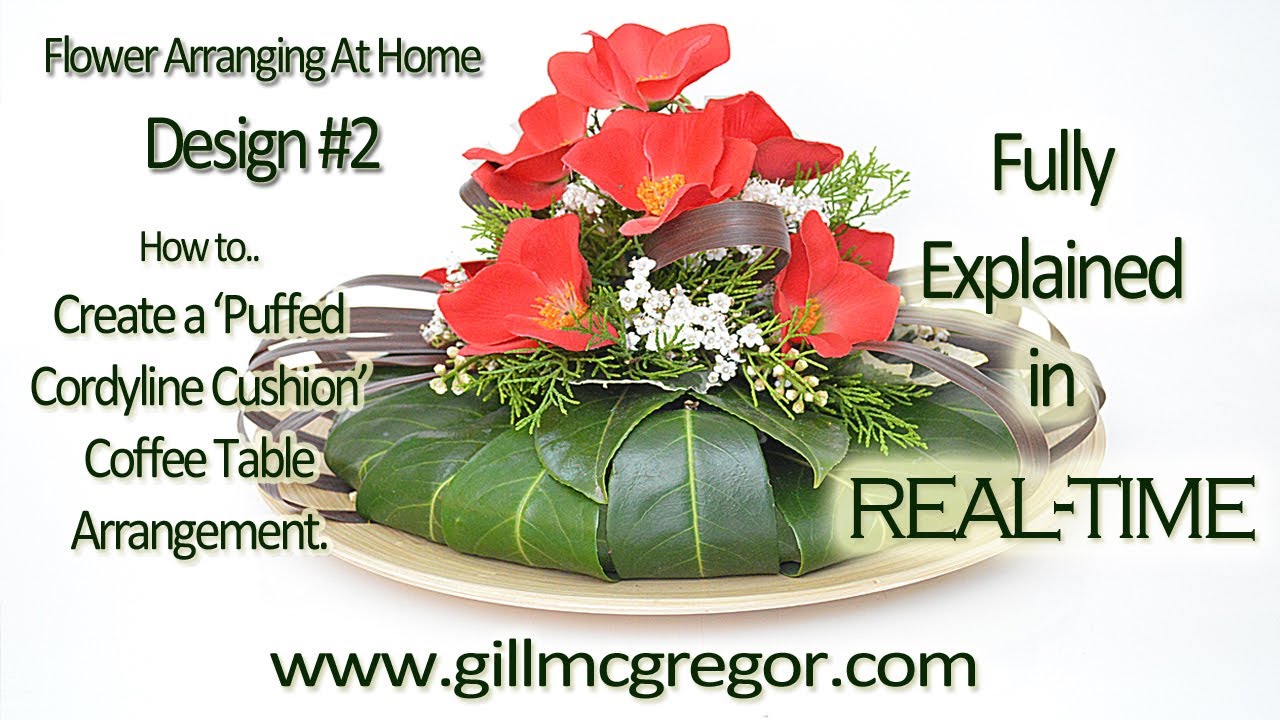The image displays a detailed flower arrangement positioned centrally and labeled with text in plant leaf green. The caption reads: "Flower Arranging at Home, Design No. 2, How to Create a Puffed Cordyline Cushion Coffee Table Arrangement. Fully Explained in Real Time. www.gillmcgregor.com." The design is set on a white plate, featuring large green leaves bent to form a lip around the arrangement. Within this leafy border, the arrangement includes some greenery with small white buds, such as lilies of the valley, and prominent red flowers with orange-yellow centers. Additionally, a silvery gray ribbon is loosely intertwined at the base, adding a touch of elegance to the design. The background features writing encircling the arrangement, explaining the design and providing website information.